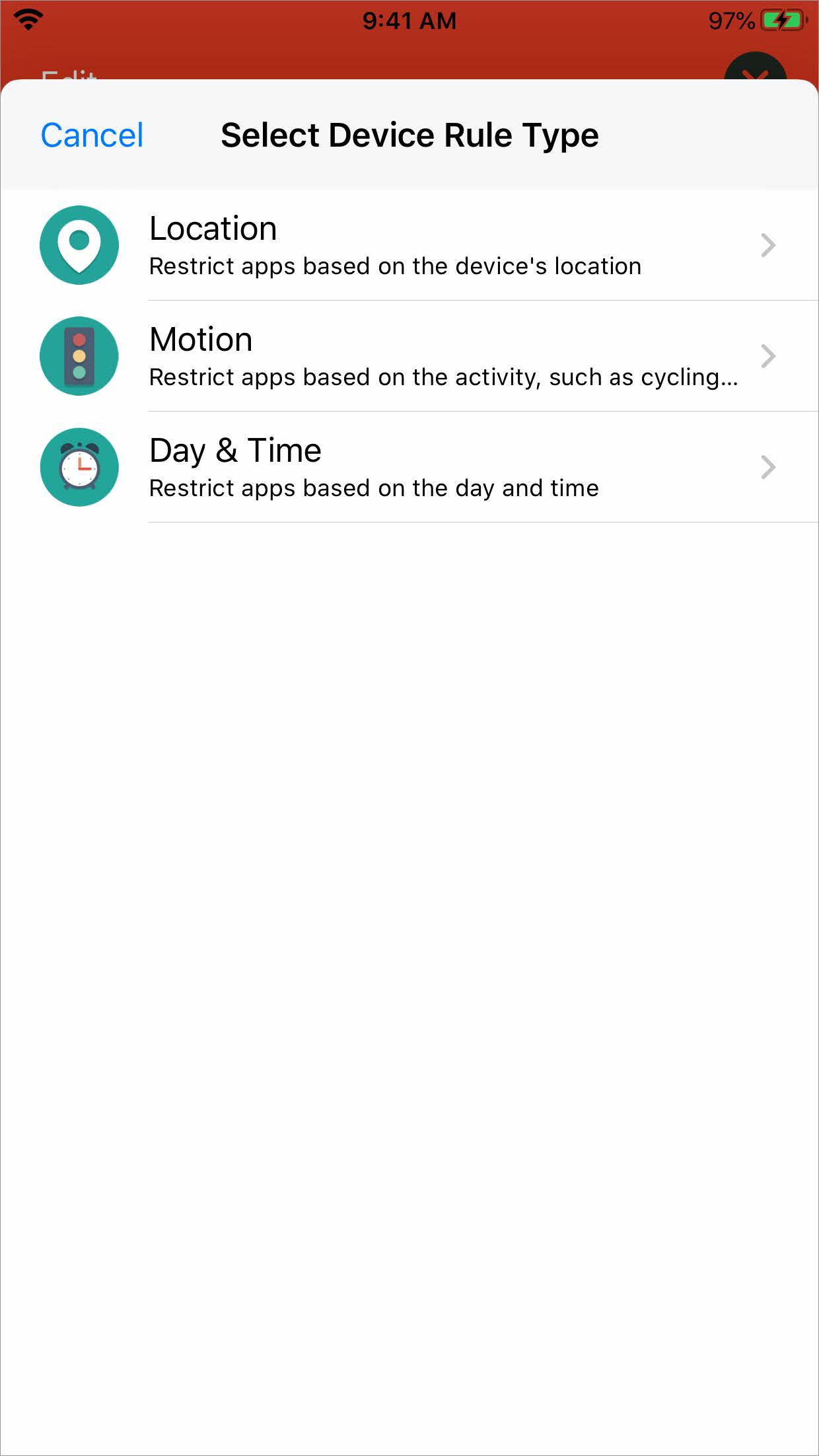This screenshot captures a mobile device's interface with several key details. At the top of the screen, the Wi-Fi signal is visible, accompanied by the current time, 9:41 a.m. The battery indicator shows a 97% charge, with a lightning bolt symbol indicating that it is actively charging; the battery icon is glowing green as a further sign of the charging status.

The device's current display is an app with a red background, featuring an active pop-up window. This pop-up prompts the user to "Select Device Rule Type" and offers three options, each with a clickable area for further details. 

1. **Location**: Restricts apps based on the device's geographical location.
2. **Motion**: Displays an icon of a stoplight, and restricts apps based on movements or activities, such as cycling.
3. **Day and Time**: Features an alarm clock symbol and allows restrictions based on specific days and times.

To dismiss the pop-up, there's a "Cancel" button available at the bottom of the window.